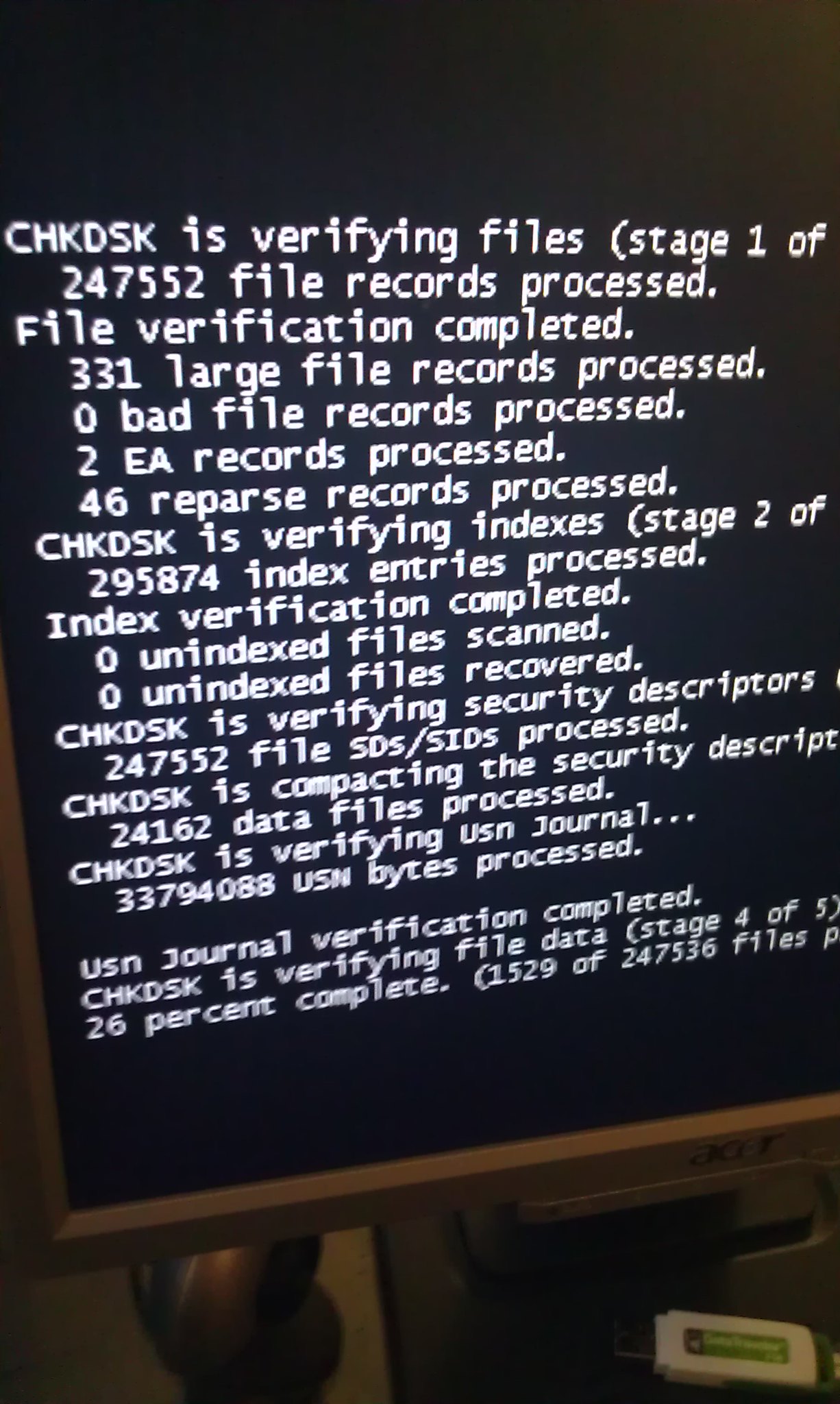The image displays a computer monitor with a black background and white text, indicative of a programming or system maintenance task underway. The screen shows a CHKDSK (Check Disk) command in progress, detailing the stages of file system verification. At the top, it reads, "CHKDSK is verifying files (Stage 1 of 247,552 file records processed)." Following this, the text indicates the completion of file verification with statistics: "File verification completed, 331 large file records processed, 0 bad file records processed, 2 EA records processed, 46 reparse records processed." The screen further shows progression through subsequent verification stages, including "CHKDSK is verifying indexes (Stage 2 of 29,587 index entries processed)," followed by the status of security descriptor checks and USN journal verification. Notably, it mentions, "CHKDSK is verifying USN journal... 33,794,088 USN bytes processed. USN journal verification completed." Lastly, it provides an update on file data verification, "Stage 4 of 5, 26% complete, 1,529 of 2,473,536 files processed." Below the screen, part of the monitor stand and a white thumb drive can be observed.